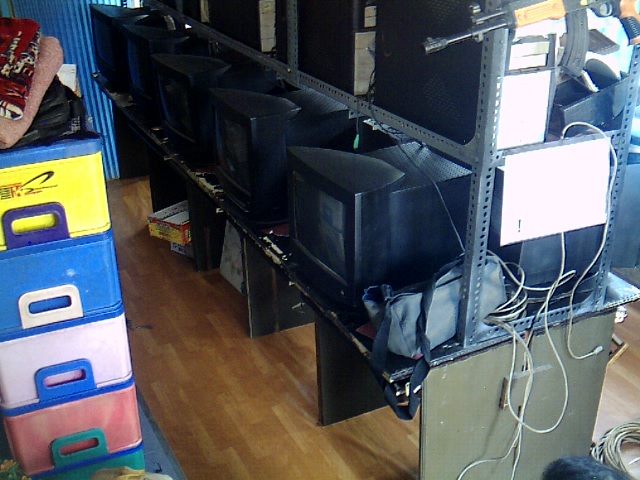The photograph depicts a cluttered storage area featuring various items on and around metal shelves. On the left side, there's a colorful shelving unit with compartments in white, blue, yellow, and light pink, topped with red blankets. Adjacent to this is a row of five old, bulky black televisions with small screens and protruding backs, all placed side by side on a dark olive-colored desk. Above the TVs on a second metal shelf, there are black-fronted devices, possibly speakers or computer towers. A light blue canvas bag with a dark blue strap and an assortment of cords hanging down are also visible. To the right, partially out of frame, hangs a toy AK-47 gun. The floor beneath is a mix of light and dark brown wood tiles. The background is filled with jumbled, indistinct items, adding to the overall sense of randomness and disorder.